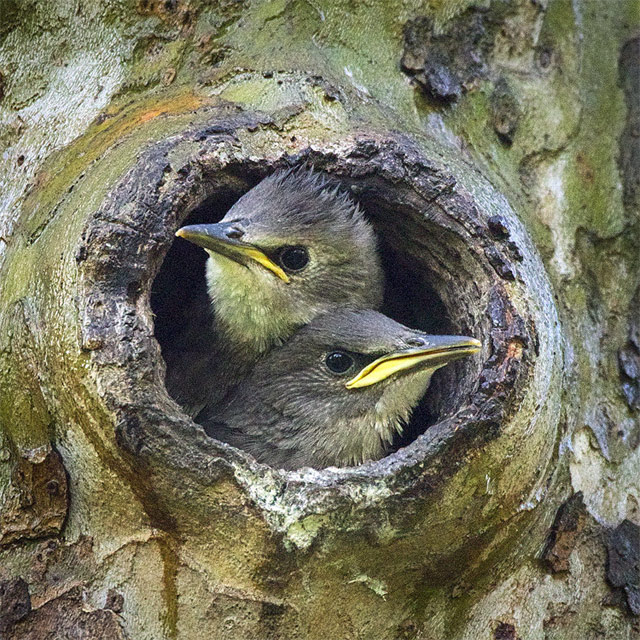A close-up image captures two small birds peeking out from a circular opening in a tree trunk, possibly their nest. The trunk has a predominantly greenish, mossy exterior, with the area immediately surrounding the hole appearing somewhat brown. Inside the dark interior of the trunk, the birds emerge, snugly positioned one above the other, almost touching. The upper bird, slightly larger and speculated to be the male, gazes to the left, while the smaller bird below, possibly the female, looks to the right. Both birds have grayish plumage with brown on their heads, dark eyes, and distinctive yellow beaks that are dark on top and white underneath. The scene is enveloped in a natural, earthy ambiance, intensified by the green moss that covers the majority of the tree trunk.